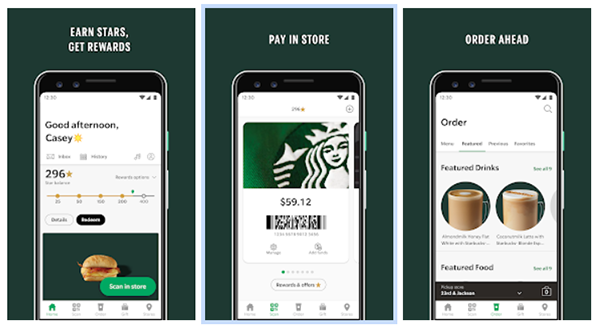The promotional display for the Starbucks mobile app showcases its functions across three meticulously designed screenshots. Each screenshot is presented on a smartphone interface set against the brand’s trademark dark green background. The trio of functionalities highlighted include: '**Earn Stars, Get Rewards**,' '**Pay in Store**,' and '**Order Ahead.**'

1. **Earn Stars, Get Rewards**:
    - The first screenshot greets the user with a personalized message, "Good afternoon Casey," and highlights the reward system, showing a total of 296 stars. It provides an option to scan in-store, accompanied by an image of a sandwich, suggesting the redemption of rewards. The interface underscores the ease of tracking and earning rewards through the app.

2. **Pay in Store**:
    - The second screenshot emphasizes the app’s payment feature, mimicking a digital Starbucks card interface. It displays a balance of $52 along with a scannable barcode for in-store transactions. A ‘Rewards and Offers’ button lies below the barcode, alongside navigation icons at the bottom, facilitating easy access to additional features and rewards.

3. **Order Ahead**:
    - The third screenshot illustrates the order-ahead functionality, presenting an order screen complete with tabs for 'Featured,' 'Previous,' and 'Favorite' items. Featured drinks such as Americano and Cappuccino, along with featured food items, are showcased with appealing images and detailed descriptions. This section promotes the convenience of pre-ordering, emphasizing the streamlined experience and reward benefits that the app offers.

Each segment cohesively reinforces the app’s ability to enhance the Starbucks experience by integrating reward tracking, seamless payment, and pre-ordering capabilities, all within a user-friendly interface.